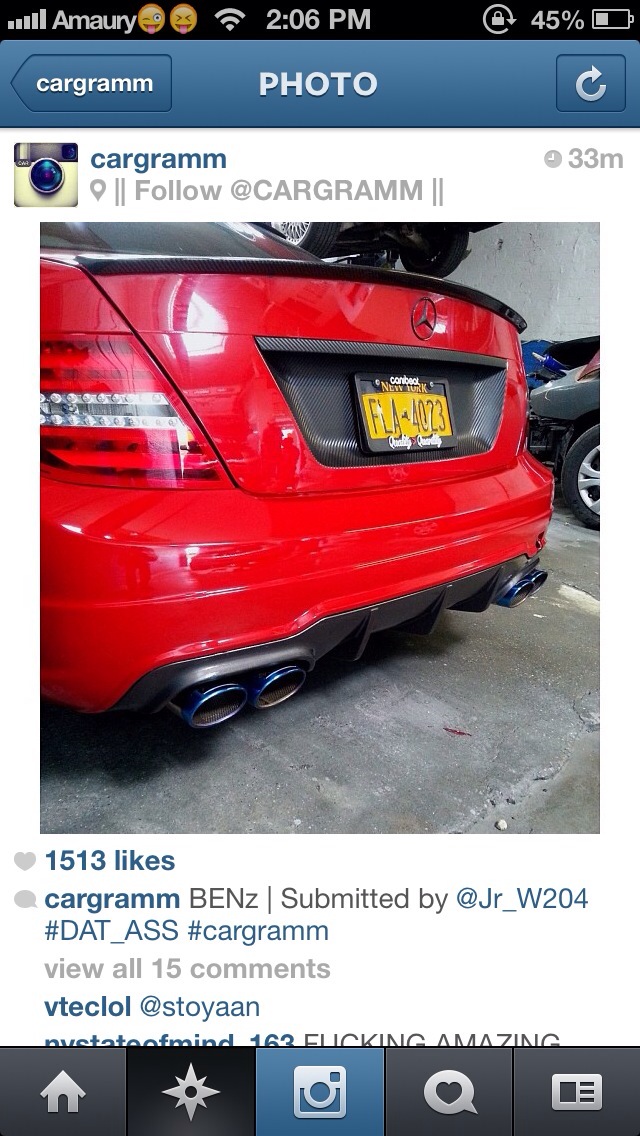The screenshot appears to be taken from an Instagram post from the account "cargram" (@cargram). It features an original Instagram interface from several years ago. The post showcases the rear view of a red Mercedes with a distinct yellow New York license plate. The car seems to be parked on a pavement within a garage setting. Surrounding the image, a blue bar displays navigation buttons including "Car Gram," "Photo," and a refresh icon. Beneath the picture, the post has garnered 1,513 likes. The caption reads "Cargram Ben's," submitted by @jr_w204, and includes the hashtags #dat_ass and #cargram. Users can choose to view 15 comments. At the bottom of the screen, traditional Instagram navigation icons are present: the home button, search button (compass), the old Instagram logo (camera), a love button (speech bubble with a heart), and an item resembling a newspaper.